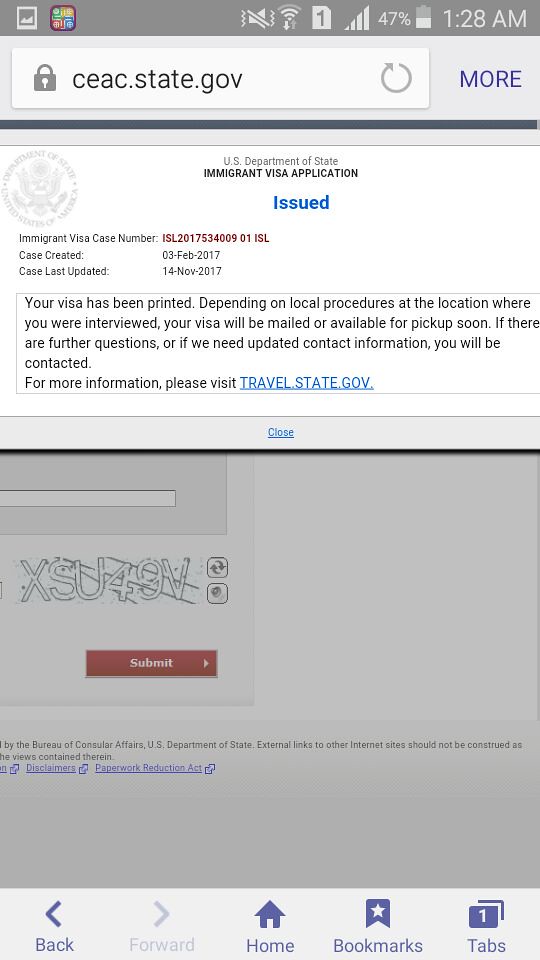This screenshot was taken from a cell phone at 1:28 AM, displaying a battery level of 47%. At the top, a gray bar shows various phone icons, including the time and battery level. Below this is the website URL, "ceac.state.gov," accompanied by a refresh button and a "More" option in blue. The main content of the screenshot is a webpage from the U.S. Department of State's Immigrant Visa Application system, prominently featuring the text "Issued" in blue. The left side of the page includes the state seal and the Immigrant Visa Case Number "ISL 201-753-400901 ISL" in red. The page details important dates: the case was created on February 3, 2017, and last updated on November 14, 2017. There is a notice in a light gray box stating that the visa has been printed and will be mailed or available for pickup soon, with additional instructions and a reference to "travel.state.gov" for further information. At the bottom of the page, there's a captcha box containing the code "XSU49V" and a red submit button. Finally, a light gray footer displays navigation buttons for back, forward, home, bookmarks, and tabs.